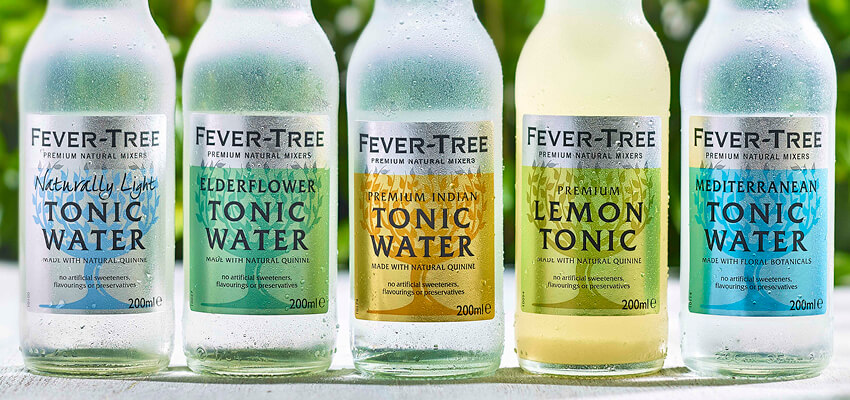The horizontal rectangular image is an advertisement featuring five bottles of Beaver Tree tonic water arranged in a row on an outdoor shelf or possibly a picnic table covered with a white tablecloth. The scene is set outdoors, indicated by the blurry green trees and leaves in the background. The close-up shot captures the bottles from the neck down, so the caps are not visible. Each glass bottle, measuring 200 milliliters, is adorned with a vertical label in different colors corresponding to the tonic's flavor, although all but one of the liquids inside are clear. The first bottle features a light blue label for Naturally Light Tonic Water, the second has a green label for Elderflower Tonic Water, the third sports a gold label for Premium Indian Tonic Water, the fourth displays a yellow label for Premium Lemon Tonic Water (which contains a yellow liquid), and the fifth bears a darker blue label for Mediterranean Tonic Water. Each silver-capped label indicates at the top in black text that it is a Beaver Tree premium natural mixer, and below it specifies either "made with natural quinine" or "made with floral botanicals." The bottles, slightly chilled as evidenced by condensation, stand prominently in the foreground of the image, inviting potential buyers to savor their refreshing contents.